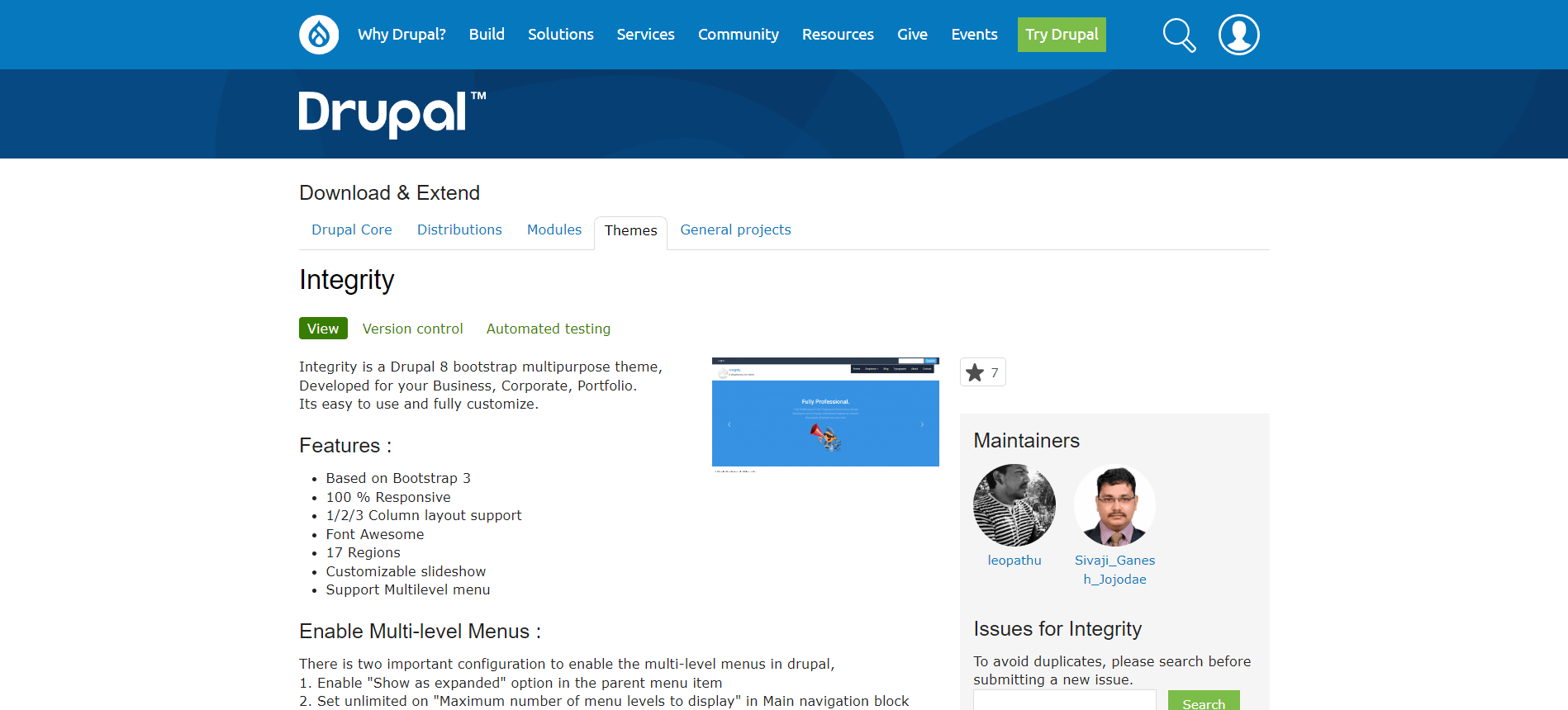**Detailed Descriptive Caption:**

The image is a screenshot of the "About" page for Drupal, a popular content management system. The page features predominantly black text on a white background, with the header bar and search area accented by two different shades of blue. At the top, the company's logo stretches from left to right. The navigation menu below the logo includes the following options: "Why Drupal," "Build," "Solutions," "Services," "Community," "Resources," "Give," and "Events." A "Try Drupal" button and a search bar, identifiable by its magnifying glass icon, are also present along with a user icon.

Beneath these elements, there is a detailed text section that explains what Drupal is, how to use it, and its various features, organized in a bullet point list. This content forms the main body of the page.

On the right side of the screen, a small menu showcases the maintainers of Drupal. It includes both a black-and-white and a color photograph of two individuals who are likely key contributors or representatives of the project.

Overall, the screenshot provides a comprehensive view of Drupal’s About page, highlighting its structure and key components, such as the navigation bar, explanatory text, and maintainers' section.